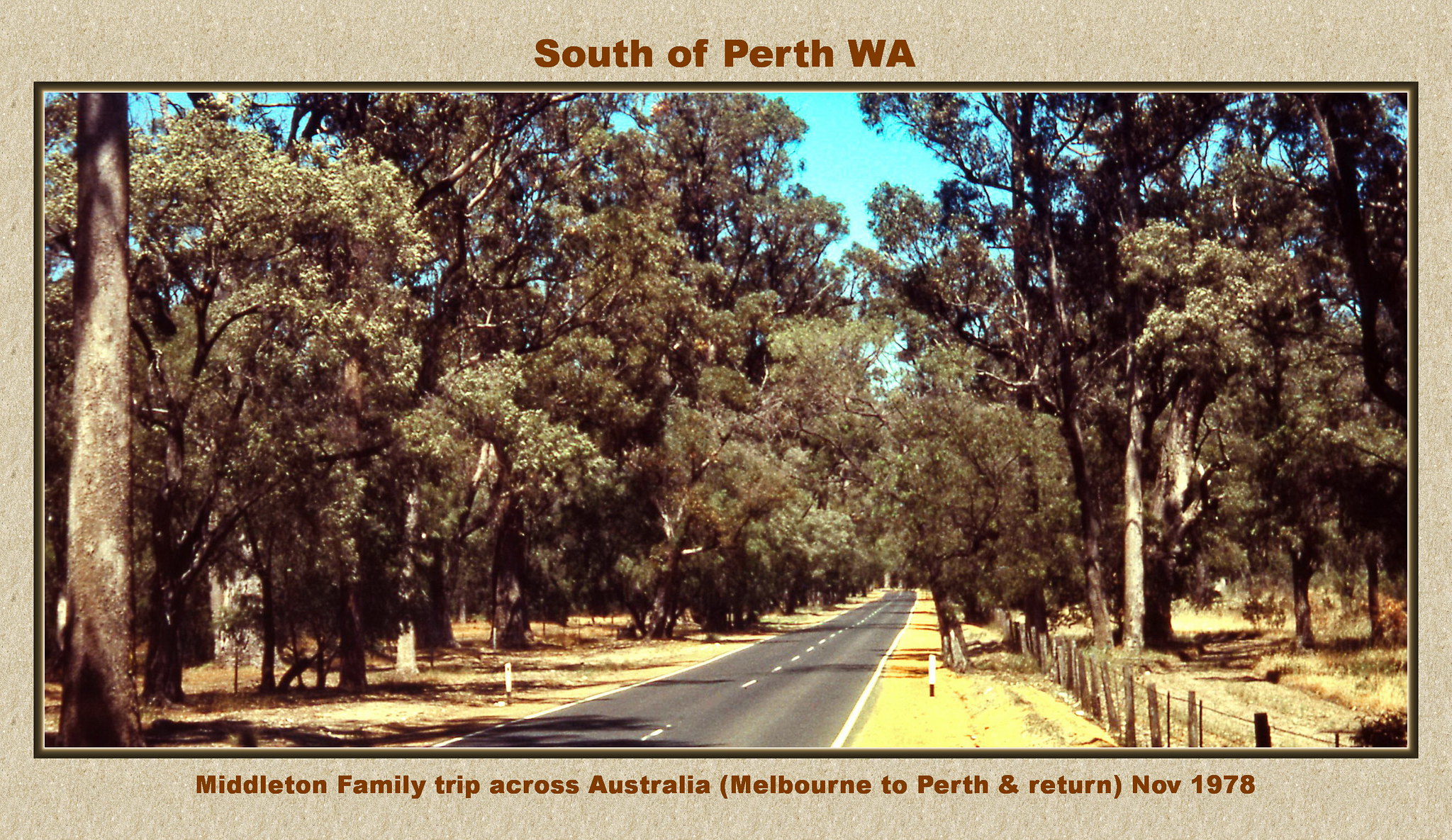The image is a color photograph, possibly a postcard, capturing a picturesque country road during daytime, lined with large, lush green trees on both sides. The well-maintained black asphalt road stretches into the distance, disappearing behind a curve. On the right side of the road, a wooden fence runs parallel, accompanied by a dirt path. There are poles with red bases and white tops marking the roadside. The photograph is inset into a slightly larger beige landscape-oriented background with dark brown text and a rule around it. The top of the image reads, "South of Perth, WA, West Australia," while the bottom caption in red font states, "Middleton family trip across Australia (Melbourne to Perth and return) November 1978." The overall style is photographic realism, emphasizing the natural outdoor setting and the orderly composition of the road and surrounding woodland.